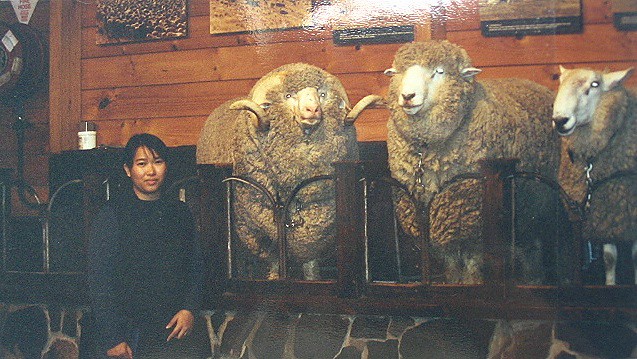In this underexposed photograph, we see a young Oriental woman standing in front of three distinct sheep. The backdrop consists of a light brown wooden wall adorned with framed pictures, partially cut off at the top. A rock wall is also visible below the sheep. The sheep vary in appearance: the one on the left has large, curved horns indicating it is likely a ram, with thick, bushy fur. The middle sheep has an unshaved head and a substantial amount of wool. The rightmost sheep has a shaved head but retains thick fur on its body. The woman is dressed in a black vest over a dark blue shirt, contrasting against the rustic wooden backdrop. The sheep are positioned in what seems to be individual stalls, possibly indicating they are in a barn or a similar setting.